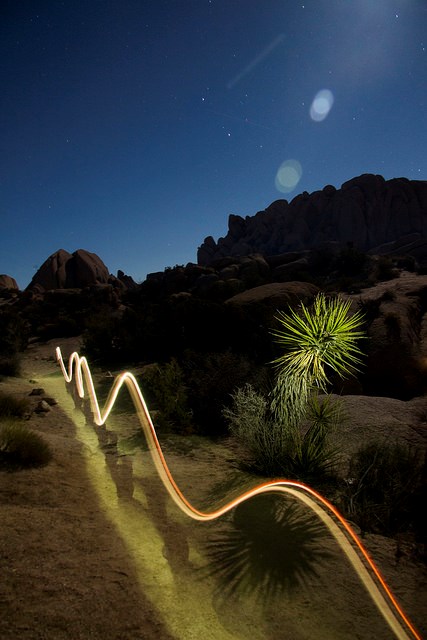In this nighttime long-exposure photograph set in a desert landscape resembling Utah, the image captures the barren beauty under a clear dark blue sky. Moonlight from the top right corner illuminates dust particles, creating an ethereal glow that enhances the scene's otherworldly feel. The moon itself remains out of frame, but its light subtly bathes the rocky cliff formations below, which spans from the left to the lower right corners of the composition.

A distinct zigzagging LED-like light traverses the hard-packed dirt path, initially appearing as a thin orange line and a wider white line. These lines form a sinuous double wave pattern, growing thicker and more pronounced as they approach the foreground. This illuminated path serves as a guide for navigation, indicative of a thoughtful trail marker.

To the right of the path, a spiky green desert plant, possibly a yucca, is vividly lit by a flashlight wielded by the photographer, drawing attention to its detailed texture against the rugged earth. Overall, the photograph masterfully conveys the serene yet mysterious atmosphere of the desert night, blending the natural and the artificial in luminescent harmony.